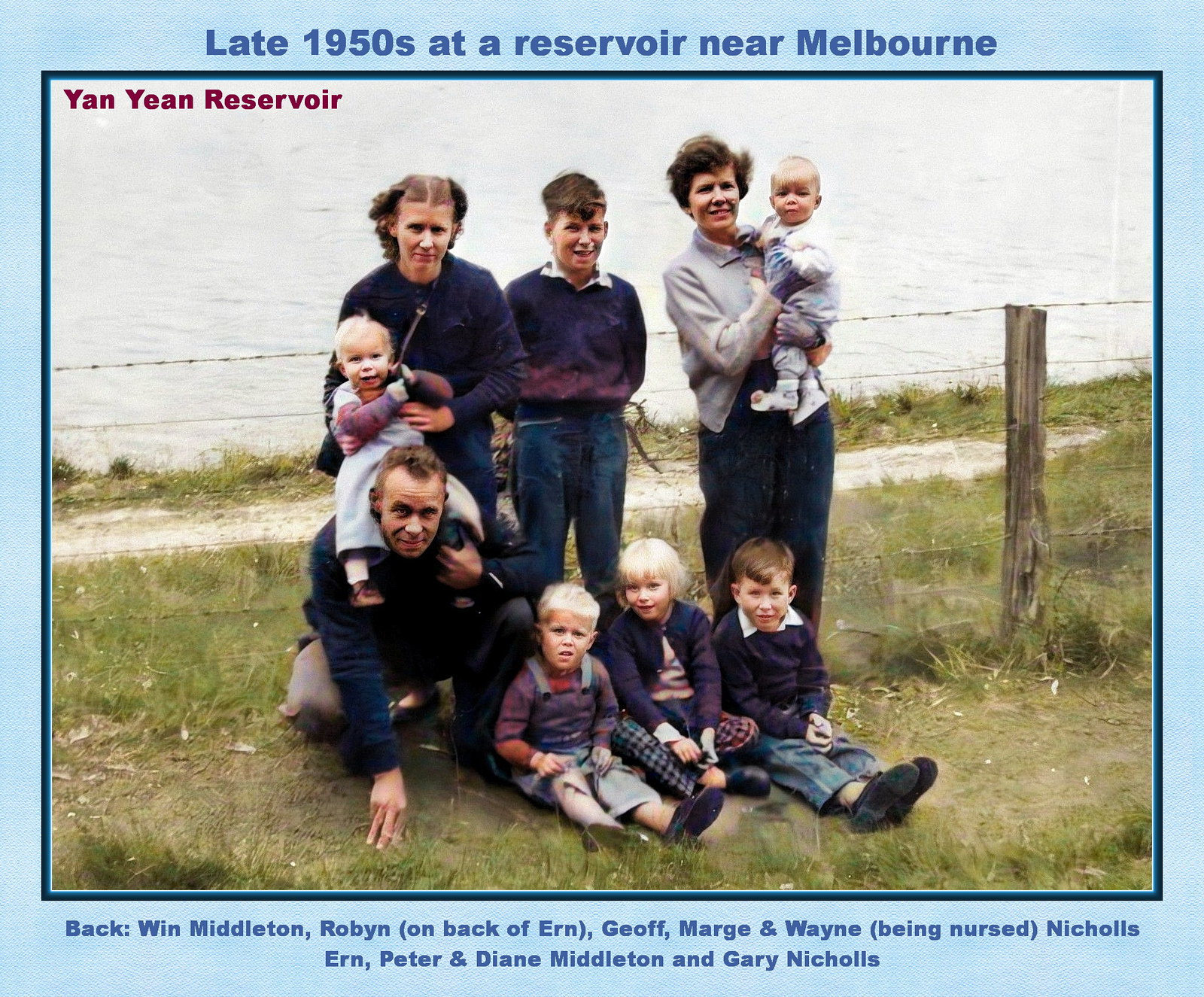This is a late 1950s photograph taken at Yanyin Reservoir near Melbourne, showing a family of nine leaning against a wire fence with water in the background. The setting appears to be chilly as everyone is wearing sweaters. The names of the family members are written in blue at the bottom of the photograph: Wynne Middleton, Robin (on the back of Earn), Jeff, Marge (nursing Wayne), Nichols, Earn, Peter and Diane Middleton, and Gary Nichols. In the image, the mother is holding a baby who appears to be about a year old, while the father, crouched with one knee on the ground, has a blonde child, also around a year old, seated on his shoulders. Three other children are seated on the ground in front of the adults, surrounded by dirt and grass.